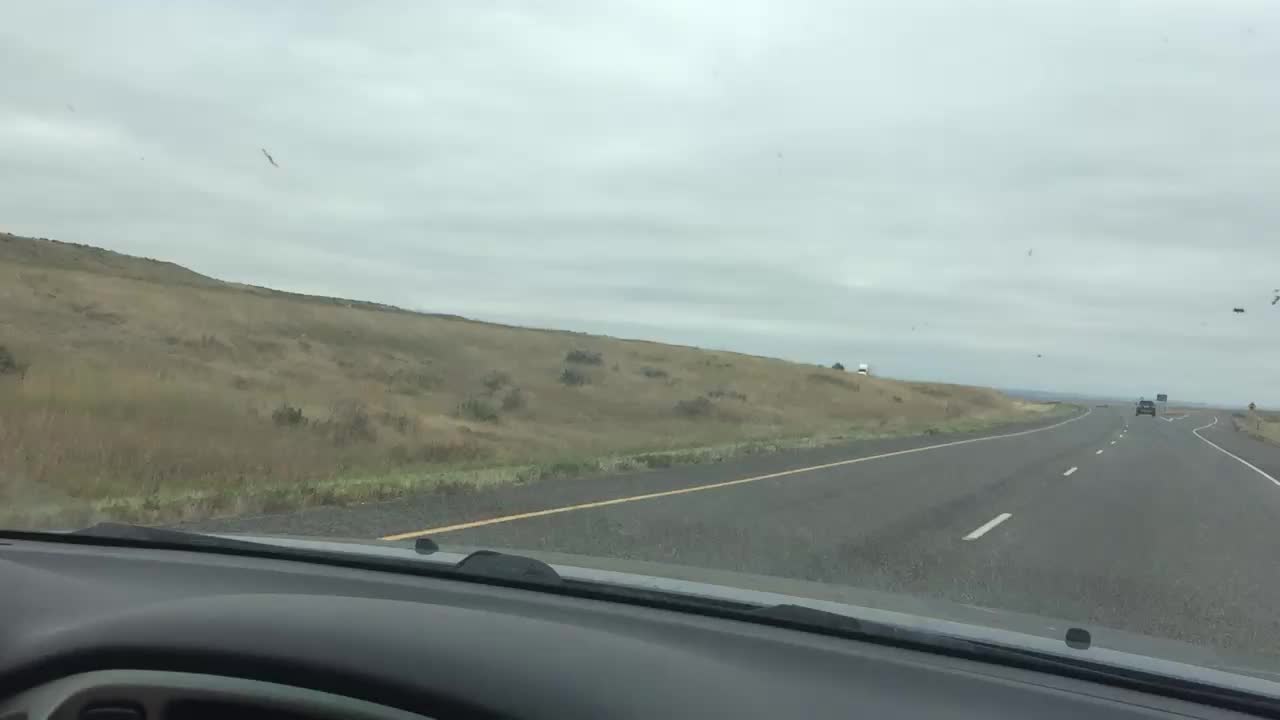Under an overcast, heavily clouded sky, the scene captures a stark contrast between nature and man-made structures. To the left lies a dry, barren field dotted with patches of parched grass, suggesting a prolonged drought or seasonal dryness. On the right, a long, gray road stretches into the distance, adorned with a series of white dashed lines that guide the way. Dominating the foreground, the view from inside a vehicle reveals a slightly grimy windshield and a plastic dashboard, adding a gritty, real-life perspective to the serene yet somber landscape outside.